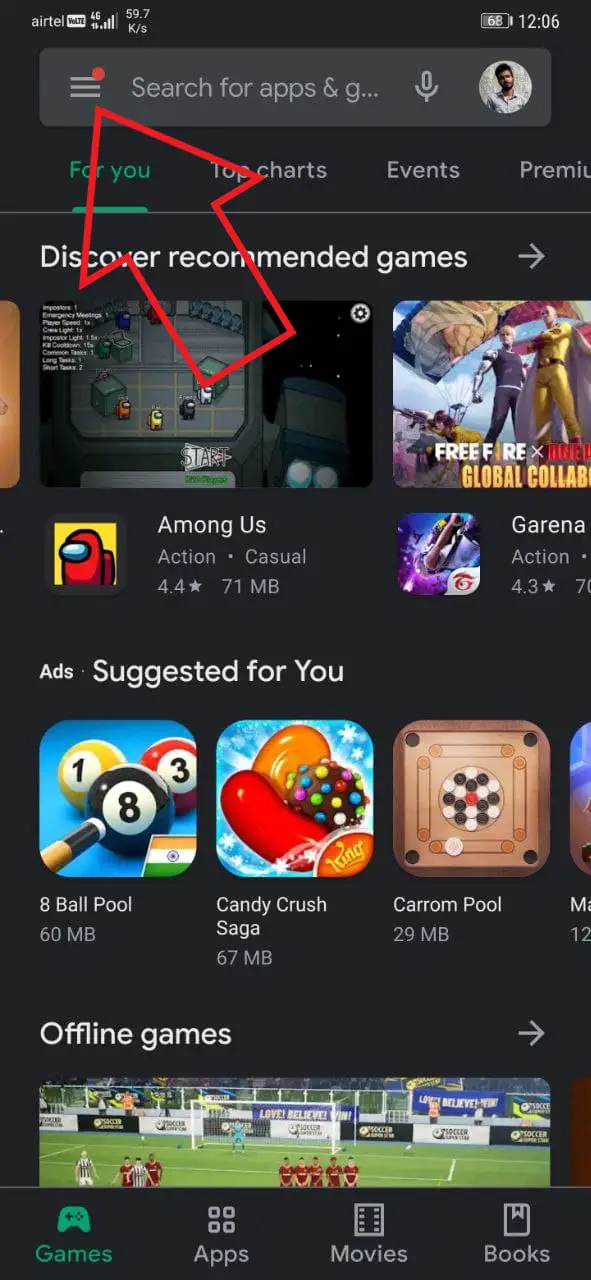This screenshot displays an Android phone screen within the Google Play Store, set in dark mode. At the top, there's a search bar featuring a user's profile picture and a microphone icon for voice search. The text "Search for apps and g" (short for "games") is slightly truncated due to the bar's limited space. A red-outlined, unfilled arrow points to the three-line menu icon within the search bar, accompanied by a small red dot.

The interface is divided into several sections: "For You," "Top Charts," "Events," and "Premium." Below this, the "Discover Recommended Games" section showcases small screenshots of games like "Among Us" and "Garena," though the full name of Garena's game is cut off. Additional sections display "Ads Suggested For You" with games such as "8 Ball Pool," "Candy Crush Saga," and "Carom Pool," followed by a partially visible "Offline Games" category.